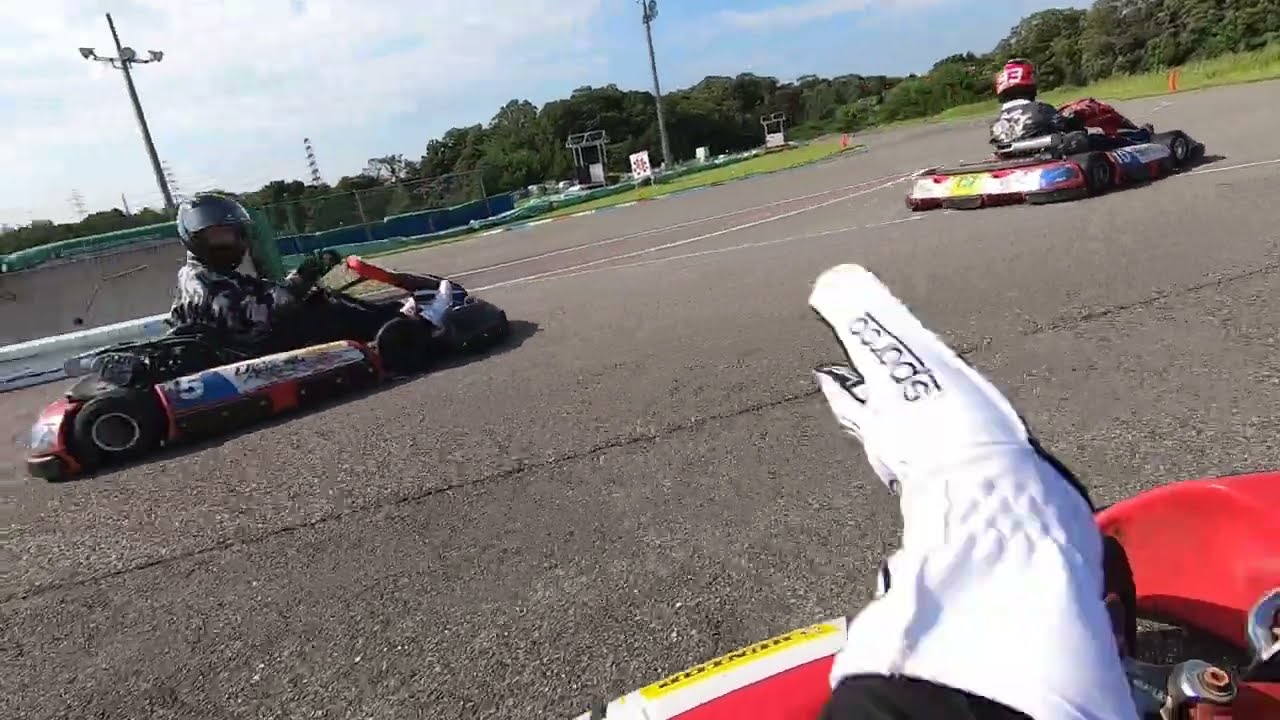In this detailed, horizontal, rectangular image, we have an action shot of a go-kart track surrounded by trees and dotted with spotlights, orange cones, and bumper markers to prevent crashes into the grass. The focus is on three go-karts in motion. Two go-karts are prominent in the top half of the image while a portion of another red go-kart, apparently without a driver, is visible in the lower right corner alongside what appears to be a white-gloved hand resting on its side.

Leading the race, a go-kart features a driver with a red helmet and a black jacket. This sleek vehicle is primarily red with silver accents and a noticeable yellow license plate area marked with the number 10. Following closely behind is another go-kart driven by an individual with a greenish helmet. This vehicle sports a red and black design with white sponsor signage and the number 5 clearly visible on its side.

The flat, low-to-the-ground design characteristic of go-karts is evident, with small tires, and vehicles barely taller than these tires except for the protruding spoilers and driver seats. The grey asphalt track curves into the distance, emphasizing the dynamic motion and competitive spirit of the scene.